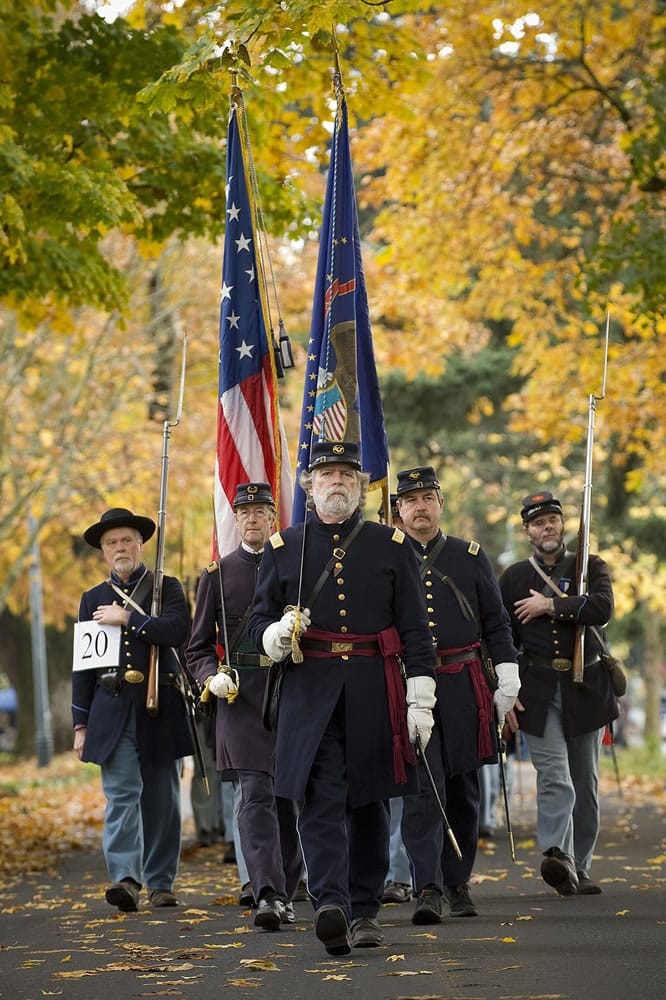The image displays a group of six Civil War reenactors, dressed in Union uniforms adorned with dark blue jackets, gold buttons, and caps, some accentuated with red tassels and gold shoulder pads. They are marching down a modern asphalt pathway, possibly in a park, set against the vibrant backdrop of autumn foliage with yellow and green trees, and fallen leaves on the ground. The reenactors carry long rifles equipped with bayonets and are organized in a triangular formation, led by a single individual. Notably, two men carry flags: one bearing an older version of the American flag with thirteen stars, and the other flag's design is obscured. Three of the men wear white gloves and have their left hands placed over their chests as if performing the Pledge of Allegiance. A unique detail is a laminate with the number "20" worn by one of the men, reinforcing that this is a contemporary reenactment.